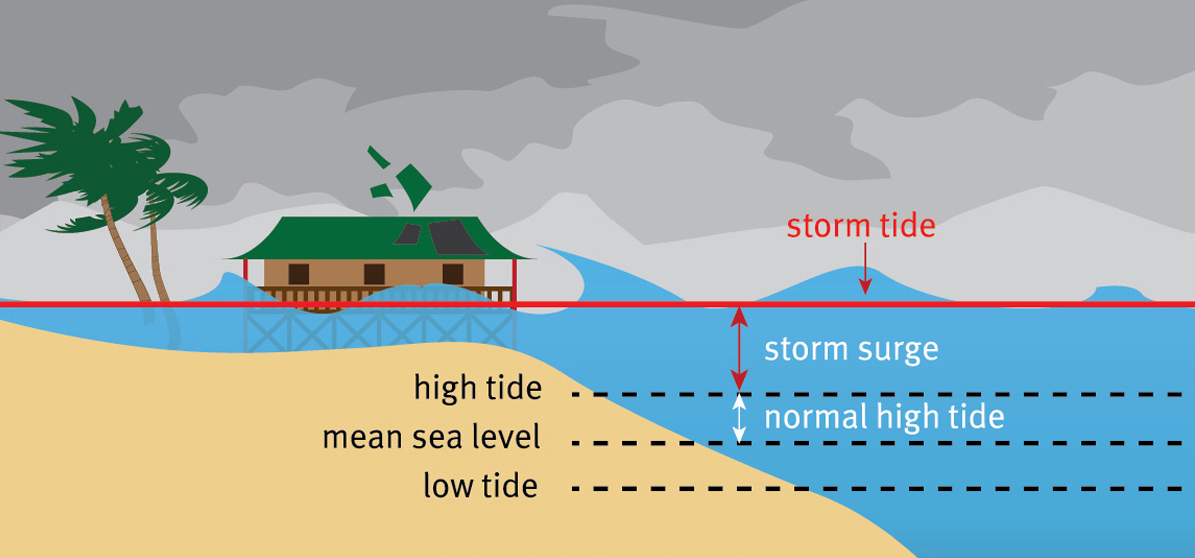The image illustrates a detailed side-view diagram of water tides during a storm. On the left side, there is a beach scene featuring a palm tree and a small wooden shack on stilts with a mansard-style green roof, which is being battered by strong winds, indicating a storm. The land slopes down towards the seabed from the left. The diagram highlights various tidal levels with significant emphasis on the storm tide, depicted by a horizontal red line labeled "storm tide" in the center. A red arrow points up from this line, indicating the storm surge. Below the storm tide line, dashed lines mark the "normal high tide," and additional text on the left side labels the "high tide," "mean sea level," and "low tide" levels in descending order. The storm tide water level is overflowing the house, with waves reaching up towards the ceiling. The sky above is dark gray with clouds, and part of the sandy beach is visible in the bottom left corner.